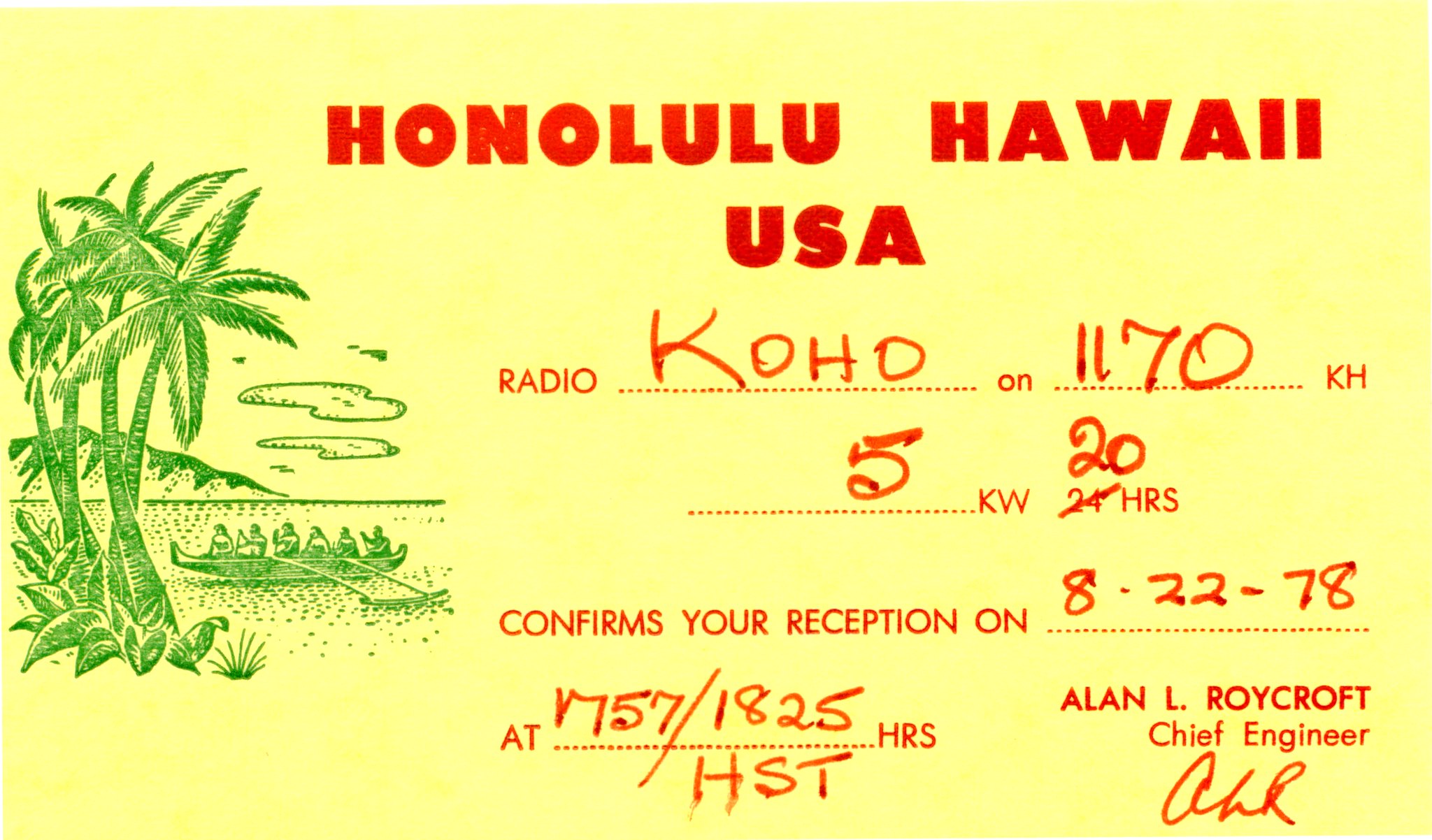This is a yellow QSL card, a form of amateur radio reception confirmation used to acknowledge communication between amateur radio operators. Dominating the left side of the card is a green graphic depicting palm trees, several people rowing a boat on a body of water, an island, and clouds in the background—evoking a Hawaiian scene. The text, all in red, prominently displays "Honolulu, Hawaii, USA" at the top. Below, it states "Radio Coho on 1170 KH, 5 KW, 20 hours," confirming the reception on "8-22-78 at 1757/1825 hours HST (Hawaiian Standard Time)." The card is signed by Allen L. Rycroft, Chief Engineer, indicating the source and authenticity of the transmission received.